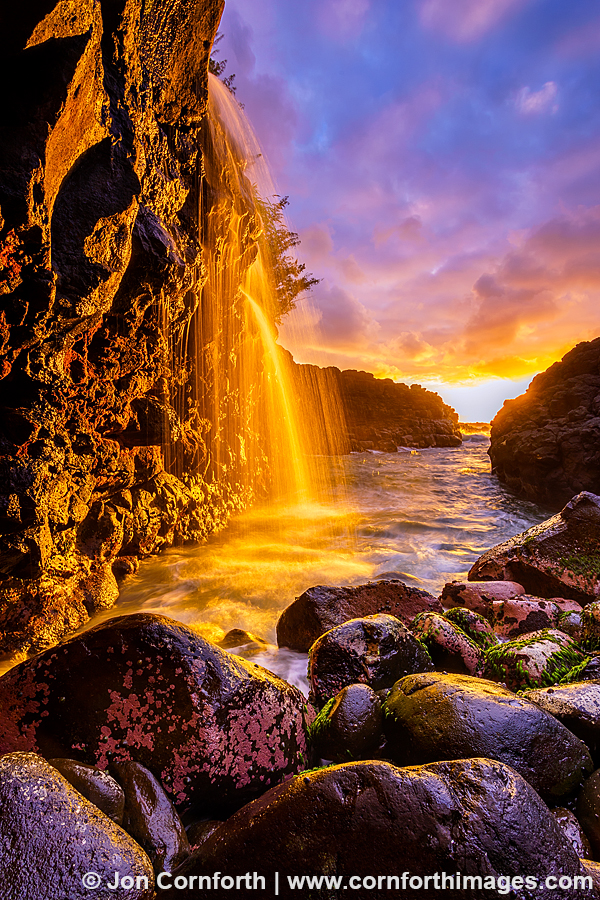The photograph captures a breathtaking, vibrant scene of a waterfall cascading from a small mountain or rocky cliff into a pool of water below, possibly leading to the ocean. The water appears to have an orange hue, potentially reflecting the brilliant and vivid sunset in the sky. Large rocks, dark gray to black in color, with speckles of red and algae in shades of pink and green, are prominent in the foreground. On either side of the waterfall are steep, rocky walls and lush foliage, enhancing the tropical ambiance of the location.

The sky transitions from a deep blue to a stunning pink and purple and culminates in a vivid orange at the horizon due to the setting sun, creating a contrast that highlights the waterfall's unique coloration. The serene yet dynamic composition is further emphasized by the dramatic lighting and the intricate details of the rocks and water. At the bottom right of the image, a white credit watermark reads "© John Cornforth," followed by his website, "www.kornforthimages.com."